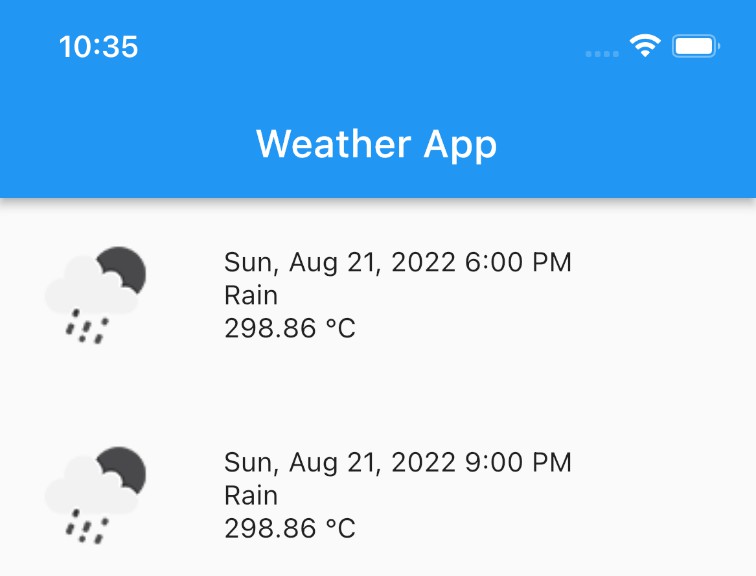A close-up screenshot of a weather app interface is displayed. At the very top left of the image, the time the screenshot was taken, 10:35, is visible. On the top right corner, the Wi-Fi and battery icons are shown, indicating the status of the device. Centered at the top of the screen, within a blue banner, the text "Weather App" is prominently displayed. Below this banner, the weather details are listed. The first entry shows "Sunday, August 21st, 2022, 6 p.m.," followed by the weather condition "Rain" and an unusually high temperature of 98.86 degrees Celsius. The next entry, which reads "Sunday, August 21st, 2022, 9 p.m.," also indicates "Rain" with the same temperature of 98.86 degrees Celsius. To the left of these entries is an icon featuring a small cloud with a dark circle, presumably representing the weather condition.